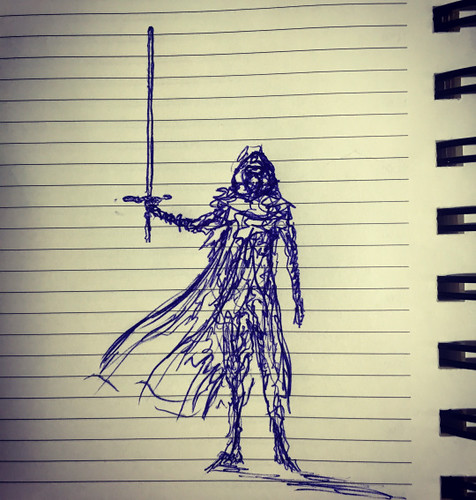This image captures a detailed pen sketch on a white, lined notepad paper. The paper is bound on the right side by black metal ring binders with square holes, indicating it's from the left-hand side of a notebook. The image shows dark blue horizontal lines closely spaced across the paper, creating the underlying structure of the sheet. The drawing, done entirely in blue pen, depicts a person facing the viewer, holding a vertically-aligned sword in their right hand. They are dressed in a cloak that billows out to the left. The figure, likely inspired by a fantasy knight or possibly Kylo Ren, is formed with dense, erratic scribbles, providing a rough but recognizable outline. The light source appears to be from the upper left, casting shadows to the bottom right of the drawing, and the figure's left hand hangs down by their side. The overall sketch is centered but positioned towards the bottom middle of the page, with no additional colors used in the artwork.